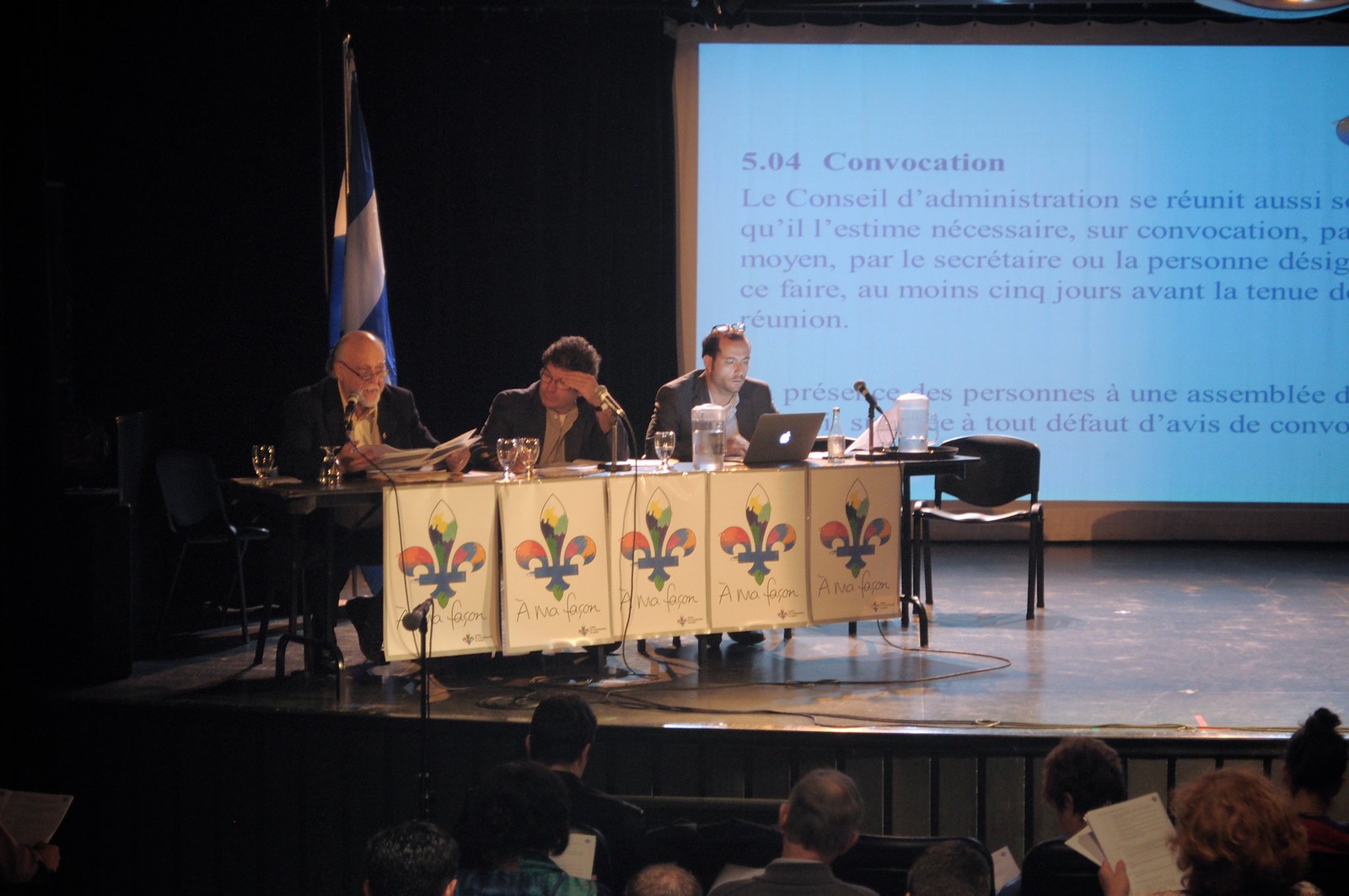The image depicts a rectangular photograph taken during a seminar or panel discussion. The event appears to be a convocation or administrative meeting, indicated by a large screen in the background displaying the words "Convocation, Le Concile d'Administration sur Renue aussi," accompanied by additional text in French. The stage features a long table to the left side, adorned with five signs featuring a floral design and black text. Seated at the table are three men, each with a microphone in front of them. 

The man on the left, a white male with glasses dressed in a black suit, is talking into the microphone while reading from some papers. In the middle, another white male with dark curly hair is wearing a gray button-down shirt with a black suit jacket and has a microphone in front of him. The third man, possibly white, Latino, or Asian, has dark hair, wears a white button-down shirt with a gray suit jacket, and is using an Apple laptop. Various items such as water pitchers, glasses, laptops, and newspapers are scattered on the table.

Behind the men, a blue and white flag is displayed. Notably, there is an empty chair to the right of the table, suggesting another person may have been present at some point. The audience seated in front of the stage can be seen at the lower part of the image, some of whom are engaged with papers. The overall setup and meticulous details indicate a formal and organized meeting environment.